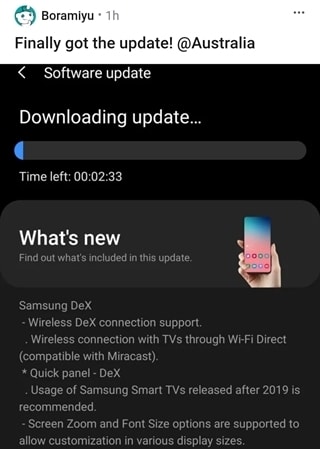In the image, there's a prominent Reddit symbol alongside a green robot, often associated with the Reddit mascot and the Android platform, respectively. Above the symbols, the username "Boramiyu" followed by "1H" indicating a post from one hour ago is displayed. Nearby, three vertical dots are arranged horizontally, suggesting additional settings or options.

The center of the image is dominated by a software update screen in progress, a common sight for Android or Samsung users. The update bar forms a gray rectangle with roughly 5% shaded in blue to indicate the current progress. Below, a timer reads "00:02:33", implying that the update is expected to complete in 2 minutes and 33 seconds. 

The update summary includes a headline, "What's New," inviting users to explore the details of the update. The background features a hand, likely a woman’s, holding a smartphone which could either be an iPhone or a Samsung device. Prominently listed among the new features is support for Samsung DeX, including wireless DeX connection through Wi-Fi Direct. The update clarifies that this feature is compatible with Miracast-enabled TVs, enhancing connectivity options for users.

Text indicating that the software update is coming to users in Australia is also present, highlighting regional availability.